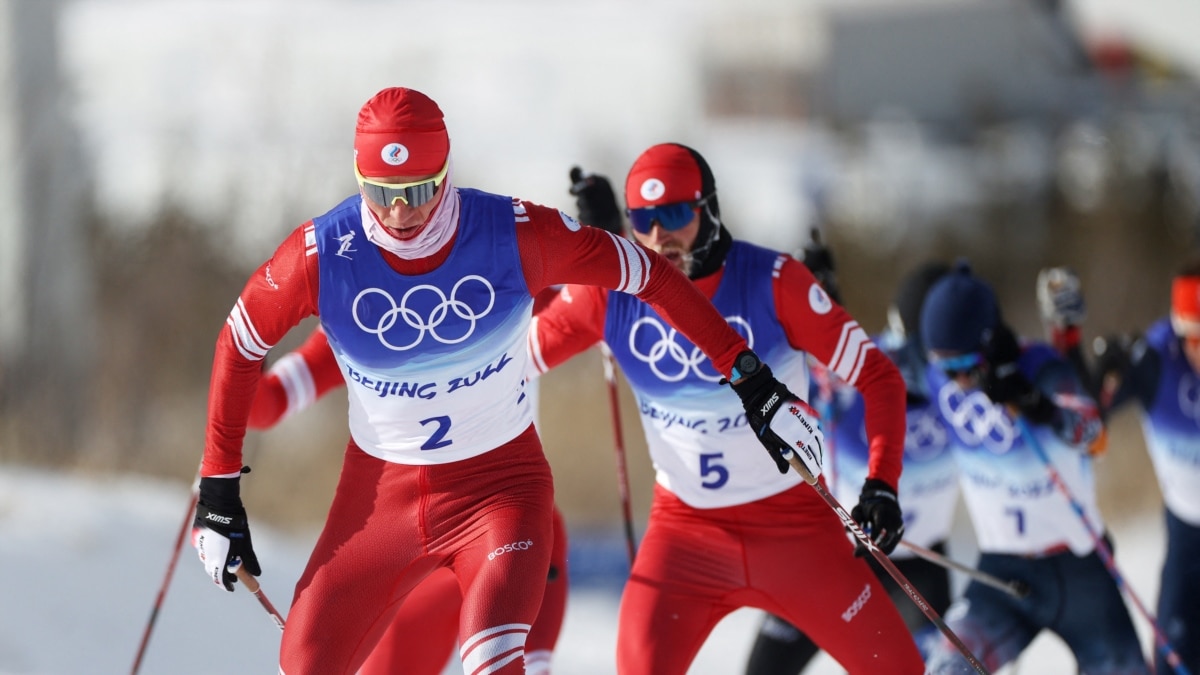The image captures a high-energy scene from the Beijing 2022 Winter Olympics, featuring a group of Olympic skiers mid-race. In the foreground, two skiers are prominently visible, clad in red bodysuits with blue vest-like jerseys adorned with the iconic Olympic five-ring logo and "Beijing 2022". The skier at the front wears the number 2, while the one behind him sports number 5. Both athletes are equipped with ski poles and gloves, along with protective ski goggles. Further in the background, blurred yet discernible, are additional skiers in black bodysuits with matching blue vests, accompanied by more skiers donning blue outfits. The number 1 is visible on one of the skiers in the background. The scene is set against a snowy backdrop, with hints of trees adding to the wintry ambiance, underscoring the competitive and fast-paced nature of the Olympic event.